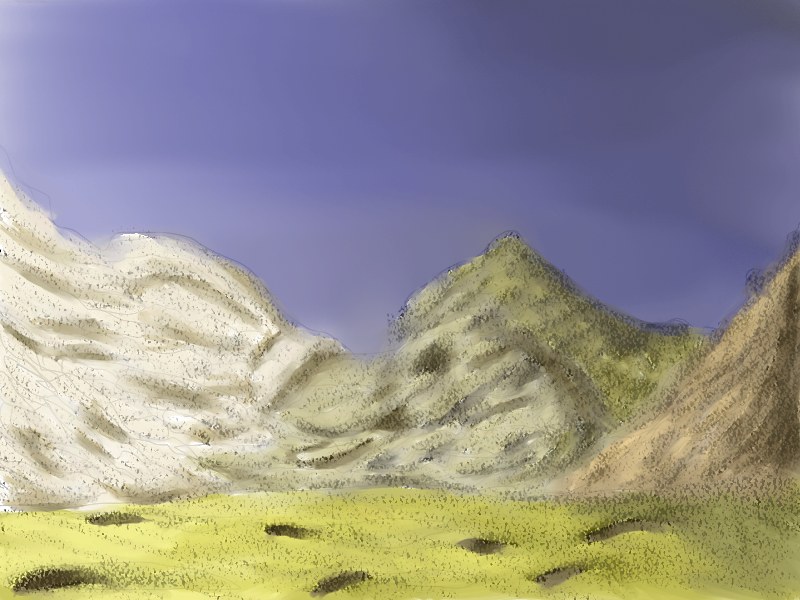A captivating landscape painting depicts a serene hill and valley scene. At the top of the picture, the sky is a soft periwinkle blue, interspersed with subtle gradients of white that gently streak from left to right. These gradients become lighter as they approach the hills below. 

On the left side of the painting, the first hill is predominantly white, accentuated with delicate brown lines that add depth and texture. The central hill is painted in a light green, matching the lush grassy areas in the foreground. The hill on the right is a rich beige, detailed with darker brown lines and specks, adding a sense of ruggedness. Scattered brown flecks throughout the hills and grass enhance the natural feel of the landscape, creating a harmonious blend of colors and textures.